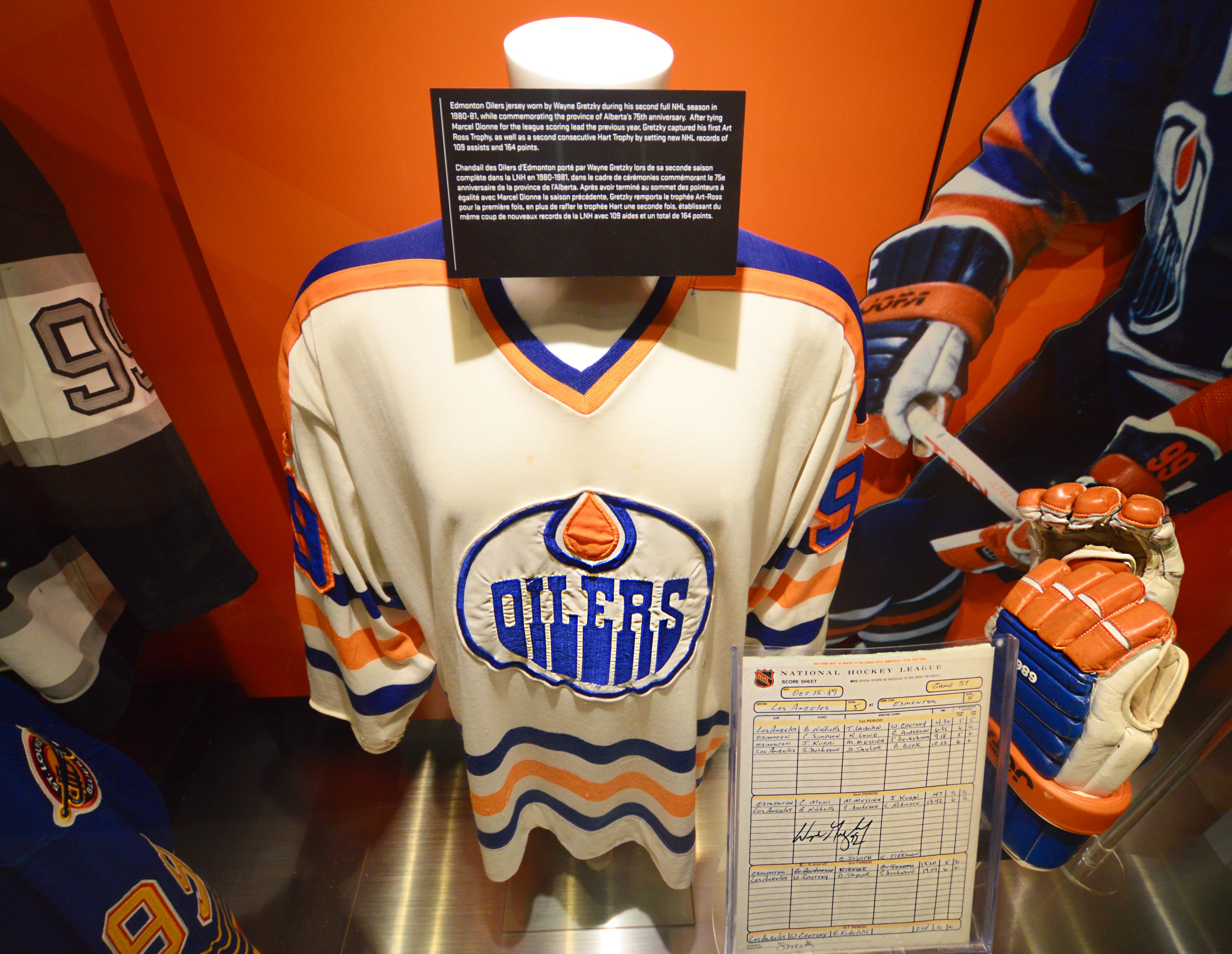The image depicts a detailed museum display featuring hockey memorabilia. Centered in the display is a headless mannequin adorned with an Edmonton Oilers jersey. The jersey showcases the number 99 prominently on both shoulders, colored in a distinct combination of blue, orange, and white, and it features the iconic Oilers logo on the chest. Situated on a shiny, metallic-looking silver floor, the mannequin is accompanied by a pair of matching hockey gloves, also in orange, white, and blue.

The background features a smooth, orange-painted wall, highlighting a photograph of the legendary hockey player Wayne Gretzky, who famously wore number 99. This photo reinforces that the jersey on display is indeed number 99. To the left of the main jersey are additional jerseys and sports equipment, hinting at more items within the exhibit, including a blue jersey with yellow "99" writing, a black jersey with white and gray accents, and another gray "99" jersey.

In front of the main jersey lies a plastic-encased handwritten note on white paper with the NHL logo and the heading "National Hockey League," though its full content is too small to read. Overall, the setting appears to be an indoor museum or exhibition space dedicated to hockey, offering a rich, immersive experience into the sport's history.